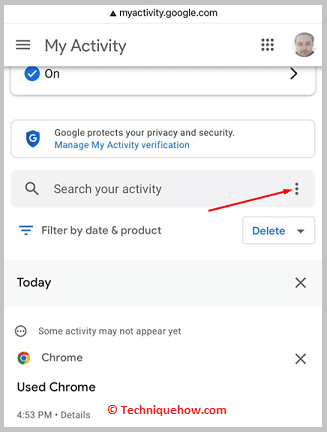Sure, here is a cleaned-up and detailed caption for the image:

---

The image is a detailed screenshot of the "My Activity" page on Google, accessible at myactivity.google.com. At the top of the page, the header features a hamburger menu on the left, followed by the "My Activity" title, and a grid icon made up of nine squares (3x3). To the right, there is a profile picture of the user with a drop shadow, followed by a toggle switch that is set to "on."

Someone has scrolled up slightly, revealing an arrow pointing to the right. Below the header, there is a Google security badge stating "Google protects your privacy and security," accompanied by a blue link labeled "Manage My Activity Verification."

Next is a search field with a magnifying glass icon, labeled "Search your activity." The user has highlighted the three vertical dots on the right in red to indicate additional options.

Below that section, there are three lines and an icon depicting three bars ascending in height, representing a filter option labeled "Filter by date and product." To the right of this filter is a blue "Delete" button, and a corresponding drop-down menu indicated by a downward-facing gray triangle.

Further down, there's a section header labeled "Today" in black text, accompanied by a close button marked with a cross on the right. Below this, there is a note stating, "Some activity might not appear yet." The next entry shows an activity with "Chrome" and a close button on the right. It indicates that Chrome was used at 4:53 PM, with a "Details" link provided.

At the bottom of the screenshot, marked in red, there is a copyright symbol "©" followed by "techniquehow.com." The entire screenshot is enclosed within a sharp, approximately five-pixel wide gray border.

---